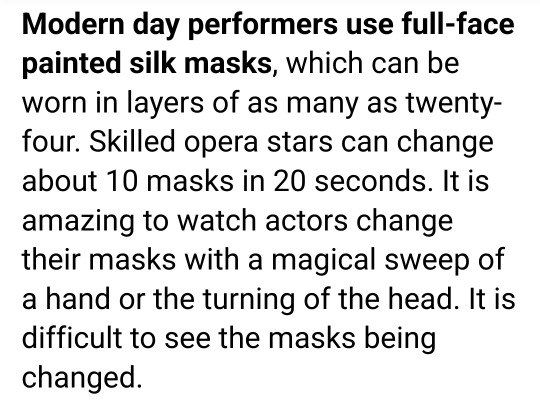The image displays a text-based paragraph against a white background with a simple, large sans-serif font in black color. The text is left-aligned and begins with a bolded phrase that reads, "Modern-day performers use full-face painted silk masks." The rest of the paragraph, which is not bold, elaborates on how these masks can be layered up to 24 at a time and that skilled opera stars can change around 10 masks within 20 seconds. It describes the mesmerizing performance where actors change their masks with a swift hand movement or a head turn, making the changes nearly imperceptible.